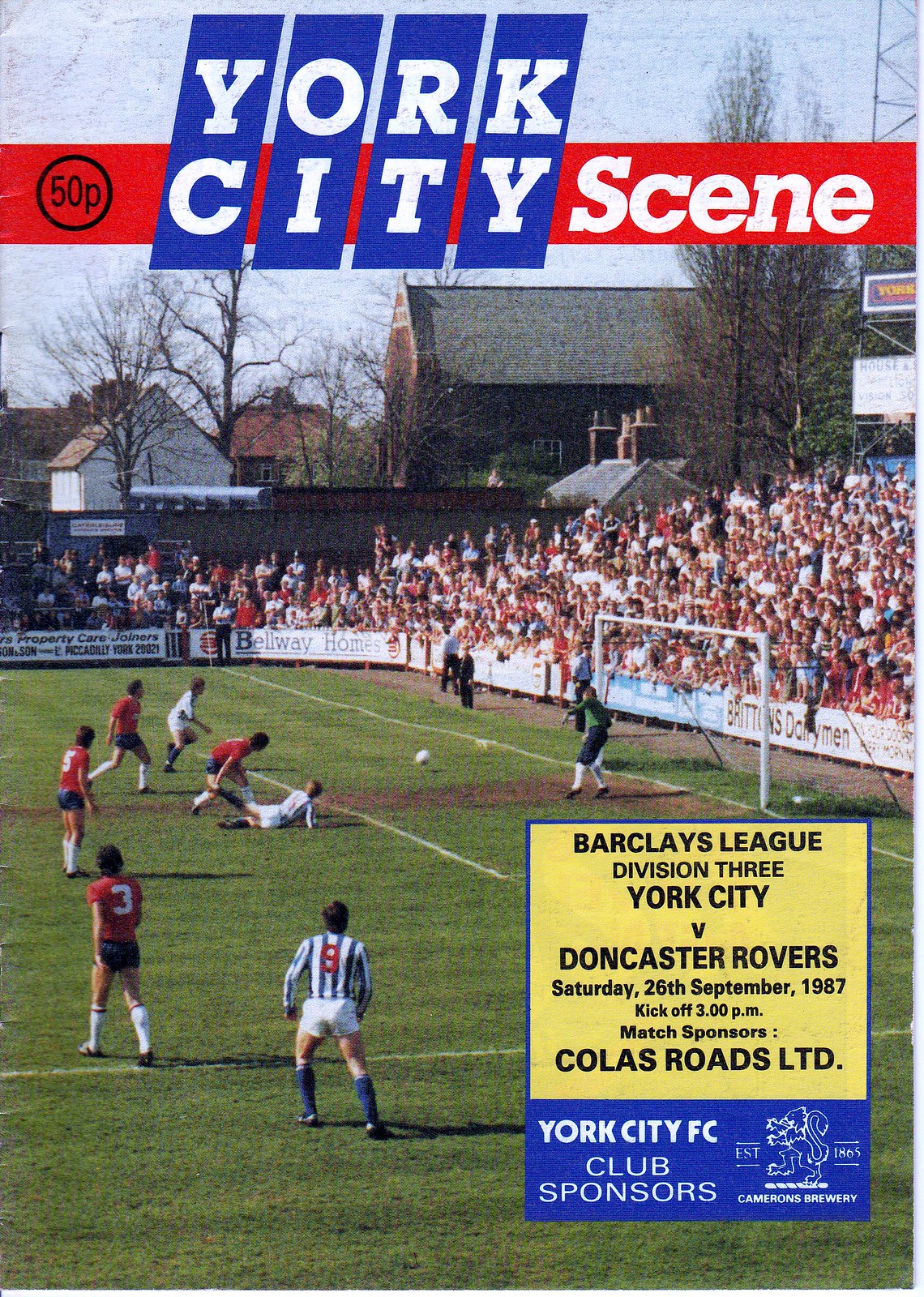The image is a detailed cover of a football (soccer) program, marked "York City Scene" at the top in white text on a red banner, priced at 50 pence. Below this, smaller blue banners with white text emphasize "York City." The main body of the cover features a dynamic scene from the match, with players from York City in solid red jerseys with black shorts, and their opponents, Doncaster Rovers, in white jerseys with white shorts. The goalkeepers are distinguished in green uniforms. The action is centered around the goal area, with an intense effort to score a goal. Behind the goal, bleachers are filled with spectators intently watching the game. An advertisement on the cover provides further details: "Barclays League Division 3, York City vs. Doncaster Rovers, Saturday 26th September 1987, kickoff 3 p.m., match sponsors Colas Roads LTD, York City FC club sponsors." The visual elements and text collectively capture the excitement and anticipation of the match day.